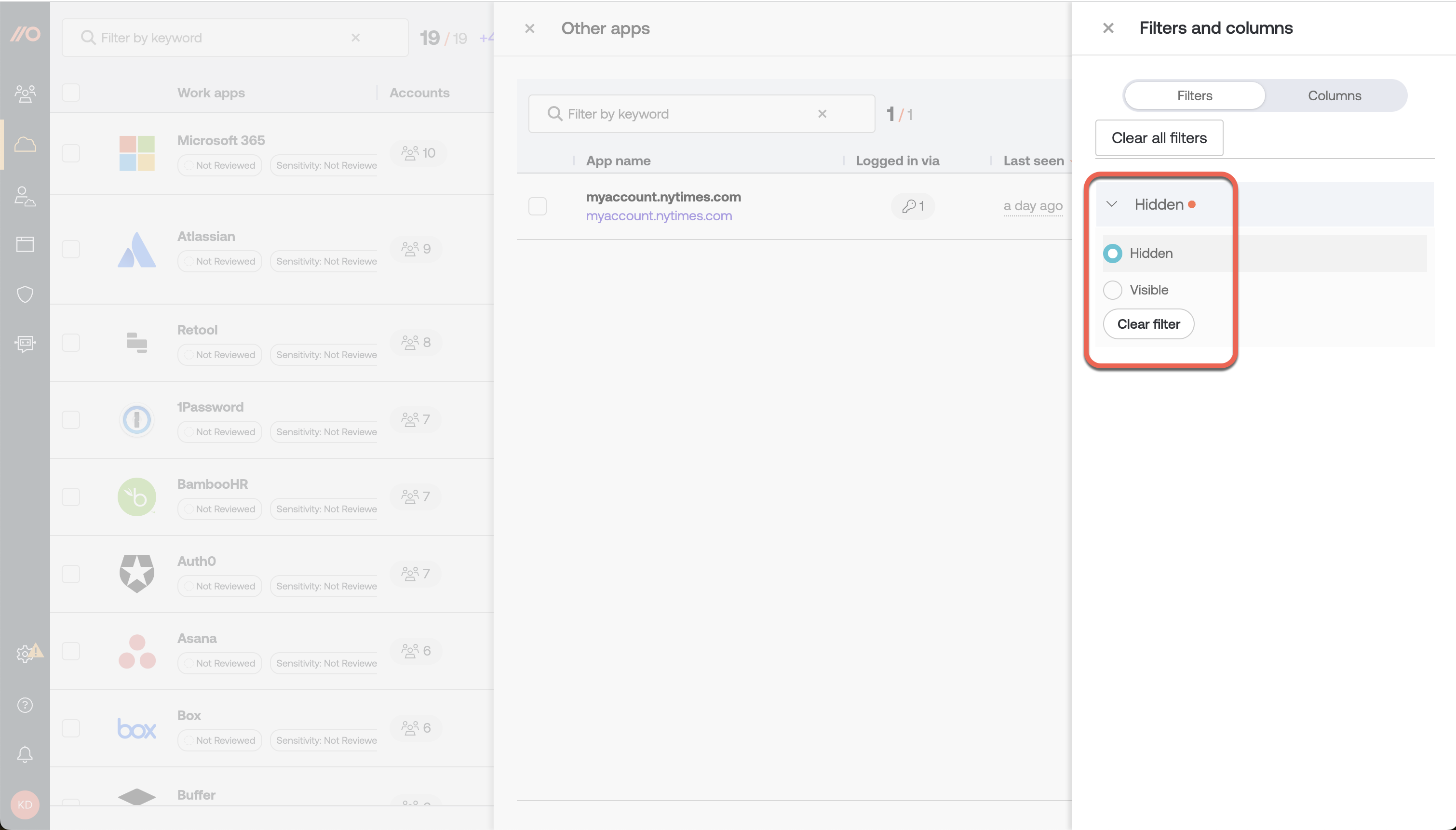This image showcases a web settings page that is predominantly grayed out, accompanied by a black navigation bar running down the left side. The navigation bar features a sequence of icons and logos, giving it a busy design. Starting from the top, the first icon resembles "slash zero", followed by icons representing people, a rock, more people, a calendar, and a shield. Further down, there are additional icons of indeterminate purpose. At the bottom of this navigation bar are icons for a cog (settings), a question mark (help), an alarm bell (notifications), and a profile circle.

In the middle of the page, there is a section with a search bar labeled "Filter by keyword". Below this, icons for various services and applications are listed, including Microsoft 365, Atlassian, Retool, 1Password, Bamboo, Auth0, Asana, Box, and Buffer. There is also a notable blank space labeled "Other apps." Another search bar is present here, likewise labeled "Filter by keyword or app name."

Further down, a section labeled "filters and columns" is visible, featuring a white button for "Filters" and a "Clear all filters" option. A highlighted tab has a red outline, indicating a dropdown menu with selectable options. The "Hidden" filter is currently selected and marked with a blue circle.